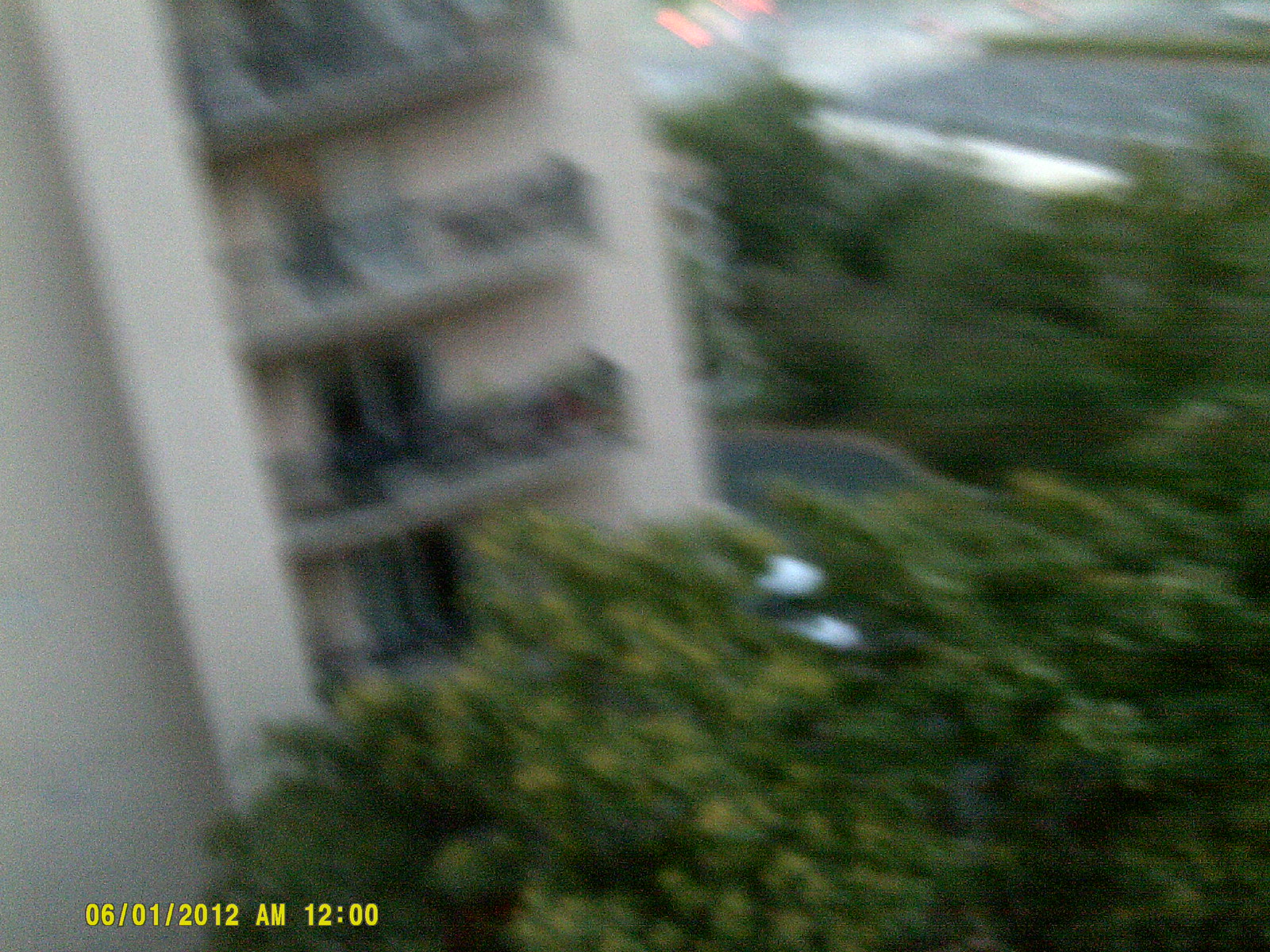This is a very blurry color photo, seemingly captured with motion blur from a point-and-shoot camera. It depicts the side of a multi-floor apartment building or possibly a hotel on the left. The building is light-colored, varying from tan to whitish beige, and features balconies on each floor. The bottom left corner of the image displays a timestamp in yellow font, reading "06/01/2012 AM 12:00." To the right of the building, dense green trees dominate the scene, with hints of a possible road in the blurry landscape. Amidst the greenery, there could be a bird with two white wings and a black body. The overall image is very hard to distinguish due to its out-of-focus nature.